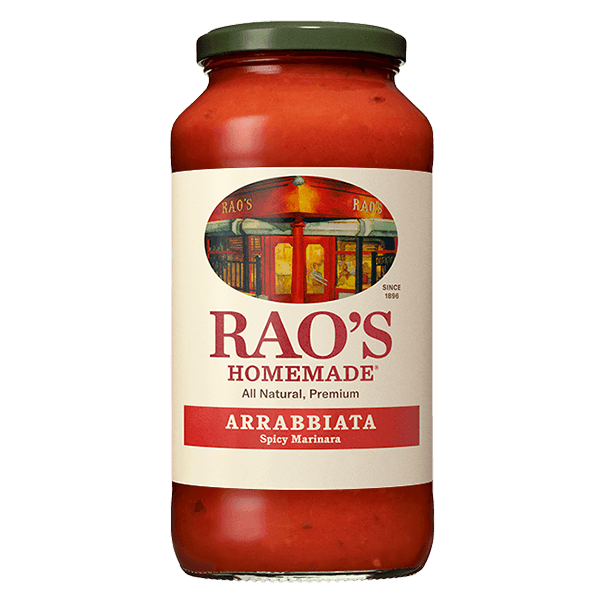The image is set against an all-white background, featuring a clear jar of RAUS spaghetti sauce prominently in the center. The jar is topped with a dark olive green lid, and the rich red sauce inside reaches up to the cap. The white label on the jar is detailed, with a central oval image depicting the entrance to a restaurant with red doors, black gates, and illuminated yellow lights, possibly illustrating the restaurant named RAUS, a premium and well-known brand since 1896. Above the image, "RAUS" is spelled out in bold red letters, accompanied by the tagline "Homemade All-Natural Premium" in smaller black text below it. Further down, a red rectangle features the text "Arrabbiata" in white, with "Spicy Marinara" written in small white letters beneath it. The label intricately blends various design elements and text to establish its premium quality and heritage.